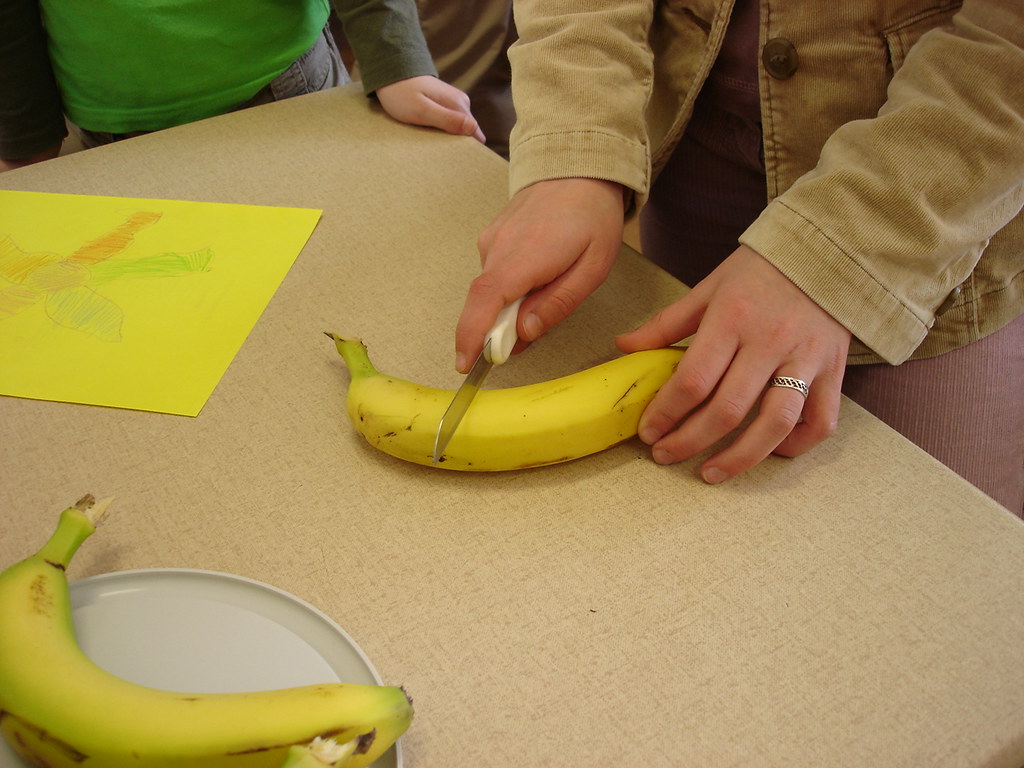In the foreground of the image, a person is meticulously slicing a banana lengthwise with a steel knife that has a white handle. Their left hand secures the banana while their right hand guides the knife, adorned with a simple ring. The individual is dressed in a brown coat adorned with matching buttons and what appears to be a blue and pink skirt. To the left, an additional, riper banana rests atop a round, gray lid. Further to the left, a vibrant yellow piece of paper displays a child's colorful drawing, featuring blue, red, and green hues arranged in a flower-like pattern. In the background to the left, a young person, identifiable by the smaller size of their hand, wears a green shirt with dark green sleeves. They rest their hand at the corner of a light beige-brown table, seemingly observing the banana-cutting process. The overall scene suggests an indoor environment where bananas are being prepared for serving.